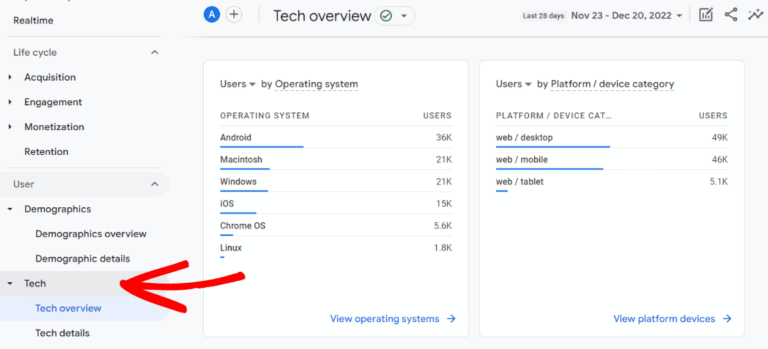**Detailed Caption:**

The image displays a web analytics dashboard against a very pale grey background, with two prominent white, page-shaped sections occupying the right two-thirds of the screen. The header at the top reads "Tech Overview of the Last 28 Days, November 23rd to December 20th, 2022," accompanied by a dropdown arrow likely intended for adjusting the displayed date range. To the right of this header are several icons for functionalities such as sharing, graphing, and an unidentified third option.

On the left side of the screen, a navigation panel lists various analytical categories: "Real Time" with several sorting options, "Life Cycle" which includes "Acquisition," "Engagement," "Monetization," and "Retention." Further down this panel, there are options like "User Menu," "Demographics," "Demographics Overview," "Demographic Details," and lastly, "Tech," which has been selected. This selection is indicated by a blue highlighted bar labeled "Tech Overview," which is emphasized further with the addition of a large, digitally drawn red arrow pointing towards it.

The left white page section is dedicated to displaying "Users by Operating Systems." This table lists operating systems in a descending order based on the number of users, including Android with 36K users, Macintosh with 21K users, Windows also with 21K users, iOS with 15K users, Chrome OS with 5.6K users, and Linux with 1.8K users. Each operating system has an accompanying horizontal blue bar that visually represents the number of users, enhancing comprehension at a glance. At the bottom of this section, a clickable blue link labeled "View operating systems" with a right arrow suggests further details are accessible.

The right white page section provides data on "Users by Platform/Device Category." Similarly organized in a descending order, this table shows user numbers for three categories: web/desktop with 49K users, web/mobile with 46K users, and web/tablet with 5.1K users. Each category includes a horizontal blue bar for visual comparison of user quantities.

Overall, the dashboard gives a comprehensive, user-friendly overview of the technological engagement over the specified period.